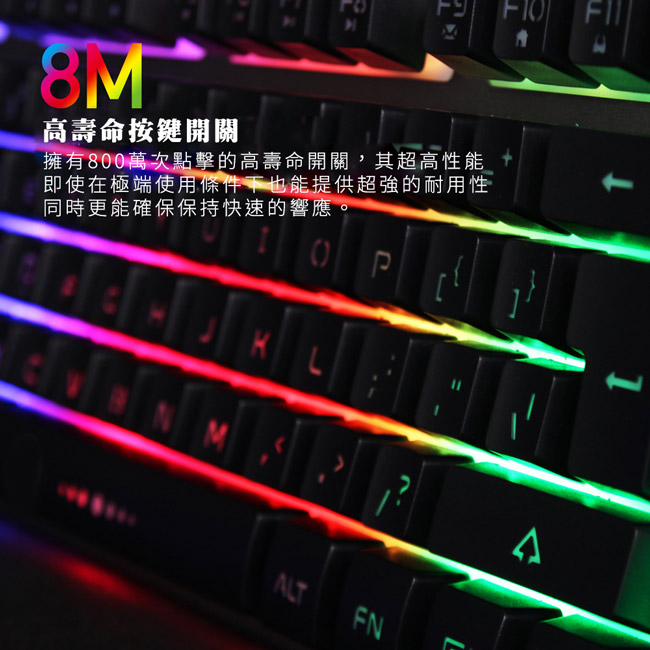This digital photograph, most likely taken indoors, features an advertisement for an RGB mechanical gaming keyboard with a prominent Chinese title and additional Chinese text below. The image showcases the keyboard's side profile, emphasizing the vibrant RGB lighting that runs through both the spaces between the keys and the keycaps themselves. The vivid color gradient transitions from dark purple on the far left, through pink, red, orange, and yellow, to green on the far right.

The keys are described as black, featuring a gamer-style font. Noteworthy keys such as the arrows, Shift, and Backspace have unique designs, with the Shift key notably resembling a pine tree. The keyboard is equipped with multimedia and macro buttons at the top, including functions for email and home.

Prominently displayed in the top left corner of the image are the characters "8M," rendered in a rainbow of colors—blue, pink, red, orange, yellow, and green. Below this, additional Chinese text includes numbers like 800800, further enhancing the advertisement’s appeal. The letters visible on the keyboard include K, L, N, M, P, and the Enter key, reinforcing its design as a dynamic and colorful gaming keyboard.